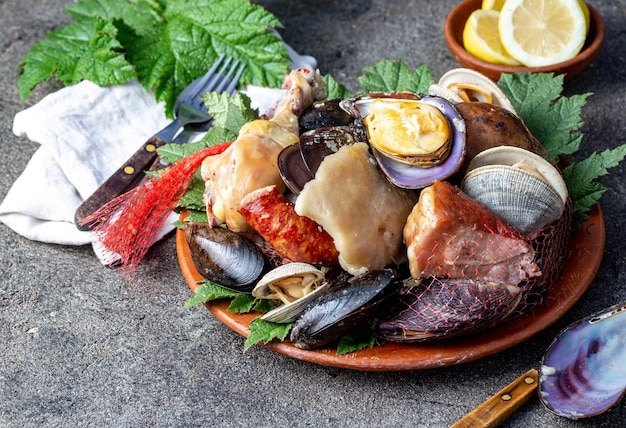The image depicts a vibrant and detailed display of seafood served on a large, round terracotta-colored plate. The plate is brimming with various types of seafood including mussels, clams, and oysters, some in opened shells and others still closed. Scattered among the seafood are larger pieces of fish, adding to the variety of textures and colors. The seafood is arranged atop a bed of green plants and red netting, providing a rich contrast in colors. To the side of the plate, a white cloth napkin is neatly folded with a fork and spoon resting on top, both featuring silver heads and black wooden handles. A knife, its handle partially visible, sits next to an empty oyster shell on what appears to be a concrete or stone surface. Additionally, in the upper right corner of the setup, there is a smaller, matching reddish-orange bowl containing slices of lemon, ready to be squeezed over the seafood. The entire arrangement exudes a sense of freshness and is visually appealing, set against the stark, gray concrete that makes the colors of the dish pop even more.